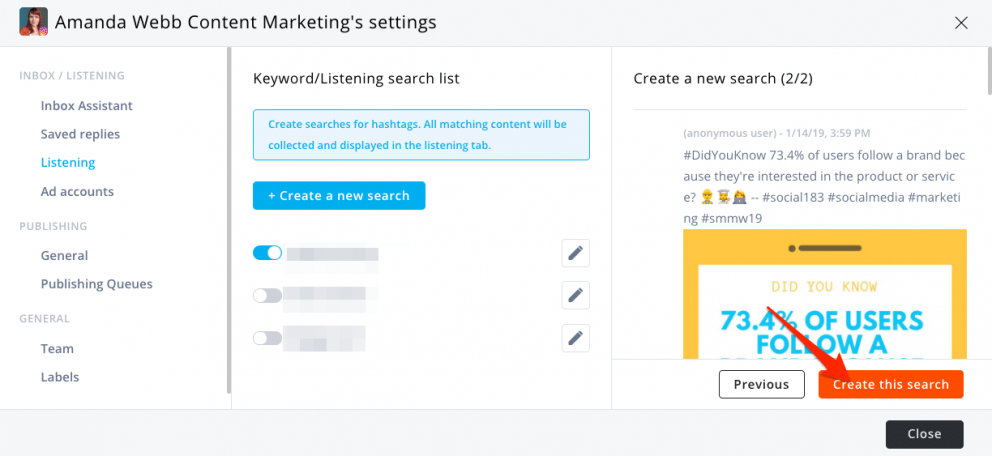The image titled "Amanda Web Content Marketing Settings" features Amanda, who is wearing a striking red jacket and has brown hair, posing against a gray background. The layout is sectioned, with a detailed sidebar on the left, a central content area, and additional elements on the right.

The left sidebar provides various navigation options, prominently highlighting "Listening" in blue. Other selections in the list include "Inbox Listening," "Inbox Assistant," "Saved Replies," "Add Accounts," and under "Publishing," options like "General," "Publishing Queues," "Team," and "Labels."

In the middle section, there's a focus on "Keywords/Listening Search List." A notable blue box encourages users to "Create Searches for Hashtags," explaining that all matching content will be aggregated and displayed in the "Listening" tab. Another blue box offers the option to "create a new search."

On the right side, images appear to be blocked out, with the first one turned on and highlighted in blue. The final column displays the directive "Create a New Search (2/2)." A yellow box with blue writing indicates that "73.4% of users follow A," where "A" is depicted as a large letter. An arrow, didactic in nature, underscores the message "Did you know?" and points to a red box labeled "Create this search," inviting user interaction.

Overall, this image intricately details the various functionalities and user interface elements available within the web content marketing settings, providing a thorough visual guide for navigating the dashboard.